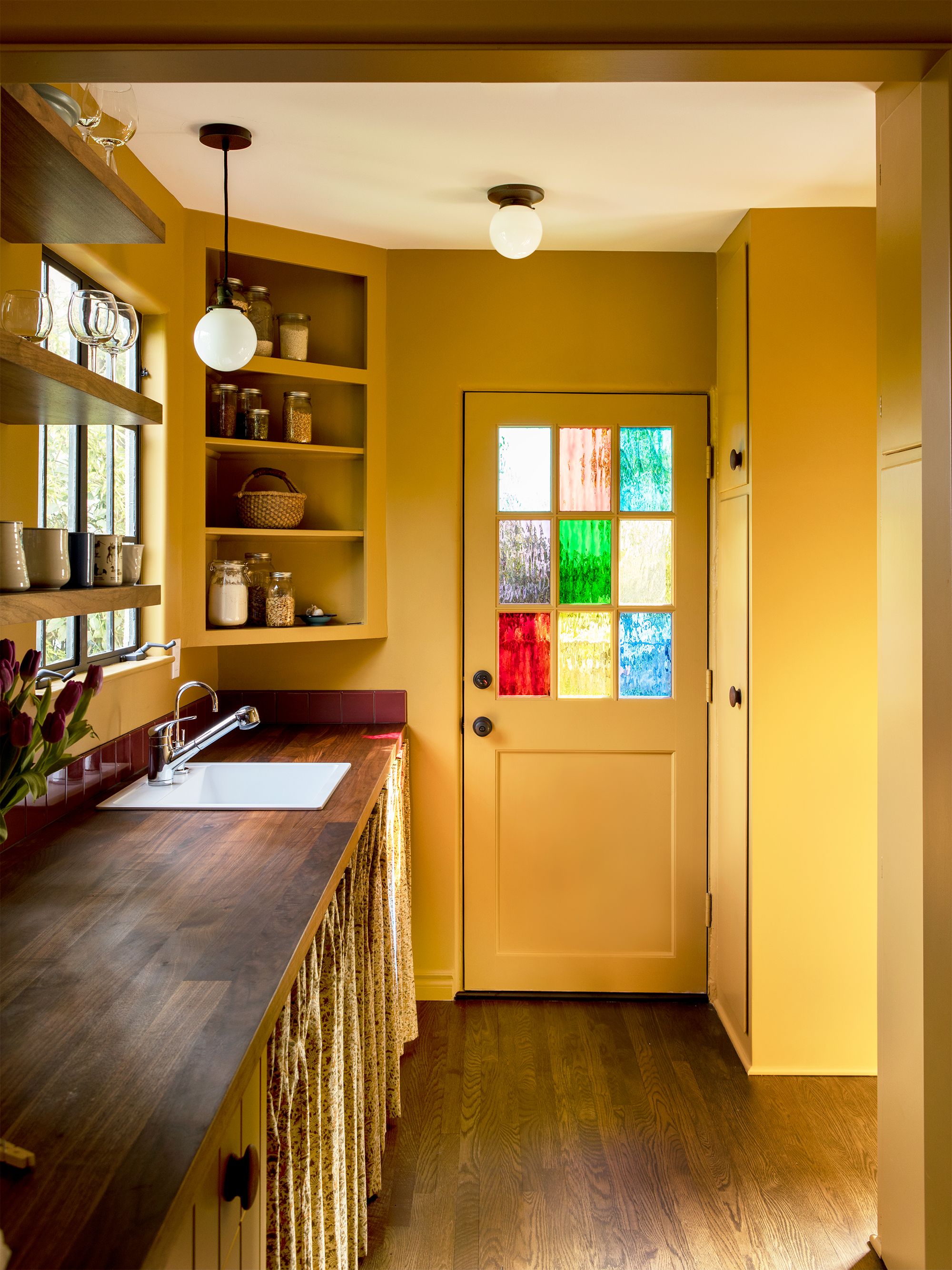This detailed interior shot showcases a bright and colorful kitchen with a dominant yellow color scheme. The kitchen features dark wood plank-like countertops and a sleek white sink equipped with a modern faucet that includes a secondary tube for rinsing. Framing the countertop is a window looking out to green shrubs, adding a touch of nature to the room. In the corner and directly beside the sink, built-in shelves display an assortment of mugs, glasses, wine goblets, and jars containing powdered ingredients and dry goods.

Above, the kitchen's lighting consists of two fixtures—a dangling pendant light and a ceiling-mounted light, both with white spherical bulbs. The room's end features a yellow door leading outside, adorned with nine stained glass panes in a variety of colors, including blue, light blue, teal, green, brown, black, red, yellow, and frosted white, which injects a vibrant, artistic flair into the space. Sunlight pours through these colorful glass panels, illuminating the kitchen and accentuating its cheerful atmosphere. Additional yellow cabinetry stands to the right of the door, extending up to the ceiling, completing the room's cohesive and bright design.